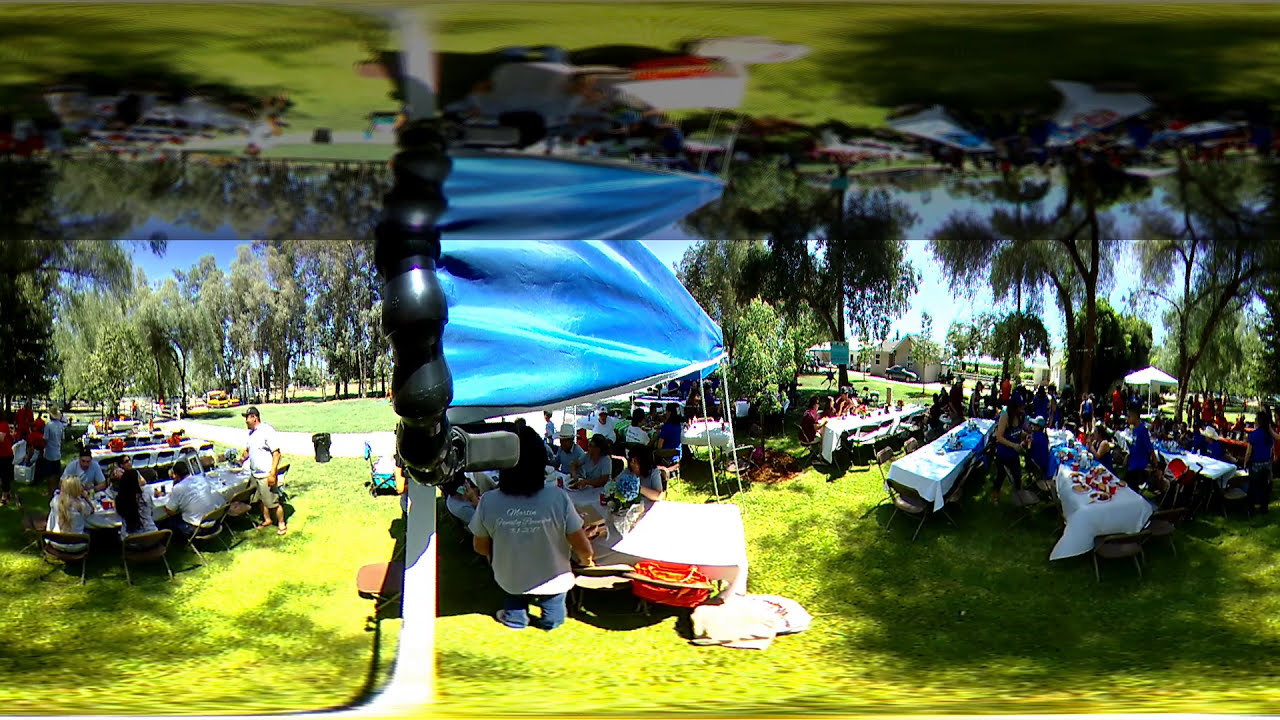The photograph captures a lively family reunion or large picnic set in a sunlit, verdant park teeming with tall trees and trimmed grass. A surreal effect graces the image; the bottom quarter mirrors the scene above, creating a reflective doubling that intrigues the viewer. This is complemented by a few warped and blended photographic elements, giving it a slightly distorted, fish-eye appearance. 

Central to the scene are long tables dressed in white tablecloths, brimmed with various foods, and surrounded by light tan metal folding chairs. At the center stands a blue canopy, shading some attendees, while similar tents dot other areas. Scattered around the tables, people, some standing and others seated, enjoy the gathering. The sky radiates a bright blue, and the lush greenery underfoot emphasizes the joyful, outdoor atmosphere of this bustling park picnic. In the background, various amenities, like walking paths and garbage cans, are visible, and the tall weeping willow trees lend shade and beauty to this vibrant community event.